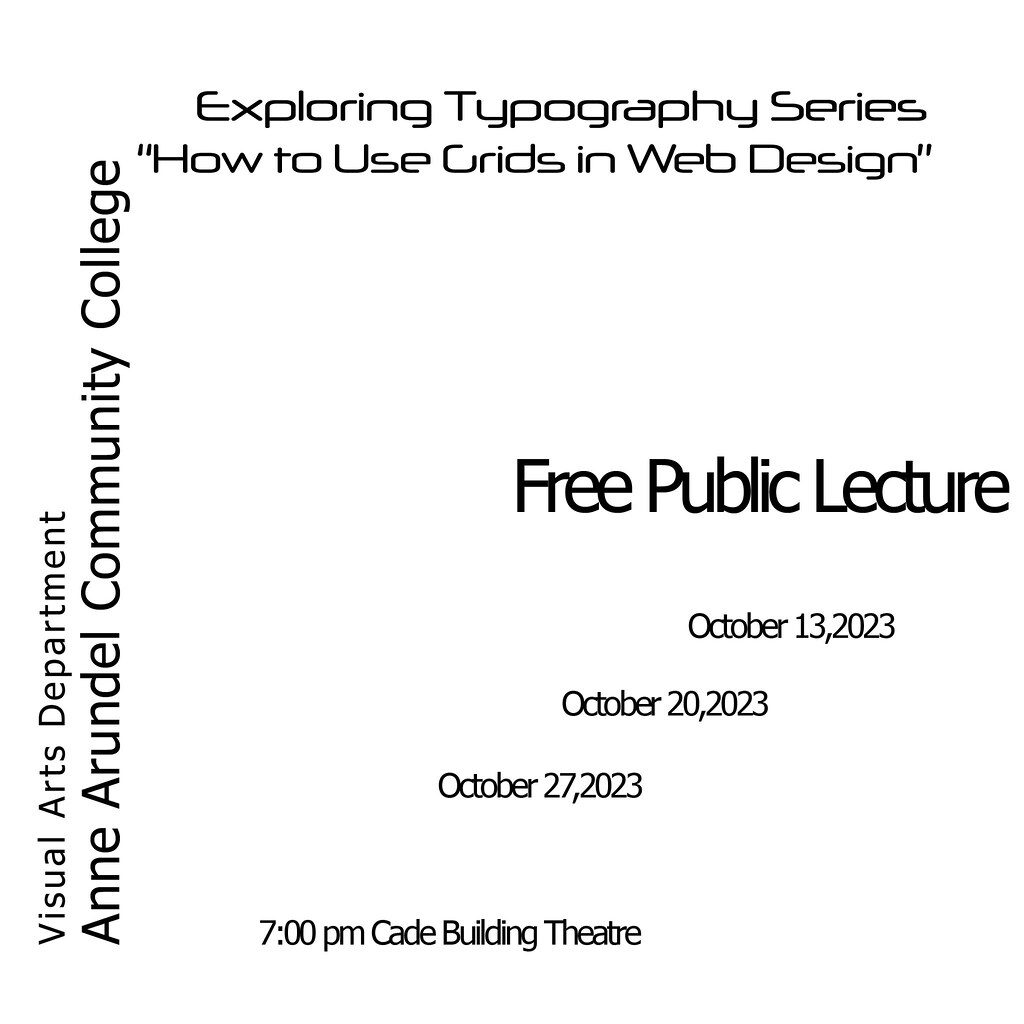The image is a black-and-white promotional poster with a minimalist design style. The top of the page features the heading, **"Exploring Typography Series,"** followed by a subheading in quotes, **"How to Use Grids in Web Design."** Along the left side of the page, the text reads vertically, **"Visual Arts Department, Ann Arundel Community College."** At the center of the page, the phrase **"Free Public Lecture"** stands out prominently in larger text.

The event details are arranged in a unique, slanted format towards the right side of the image, listing the dates and details of the lectures: **"October 13, 2023,"** **"October 20, 2023,"** and **"October 27, 2023."** Below the dates, the time and location are specified as **"7 p.m. Cade Building Theater."** The white background with the dark text gives a stark contrast, although the overall layout is somewhat unconventional and arguably difficult to read.